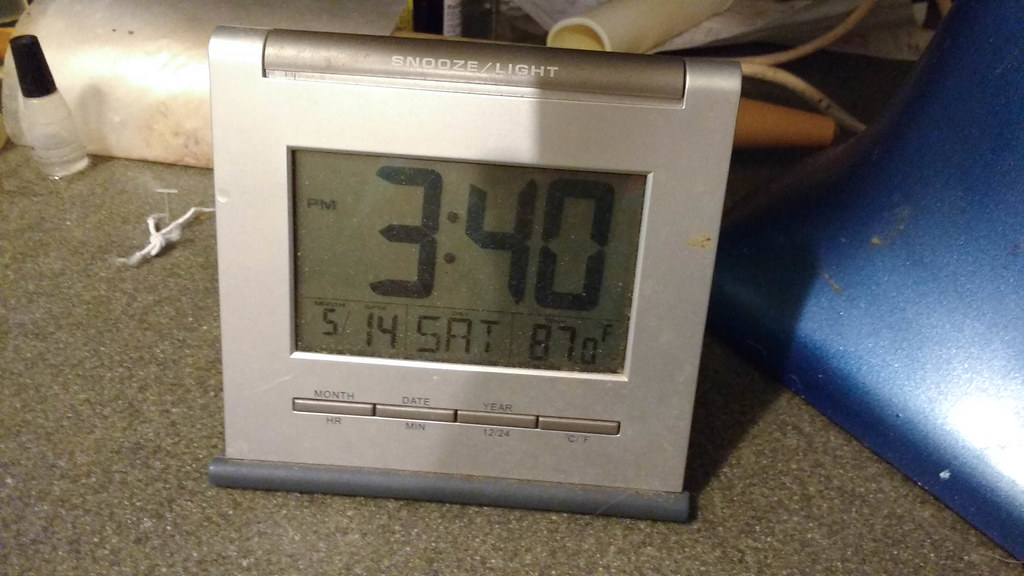The image showcases a digital alarm clock prominently displayed on a brownish granite table. The clock reads 3:40 PM on a Saturday, May 14th, with an outdoor temperature of 87 degrees Fahrenheit. The device features a conspicuous snooze/light button on its top. Below the main display are four additional buttons labeled for adjusting the month, date, and minute settings. To the right of the clock, a blue object can be seen, while to the left a silver item is partially visible in the background. Additionally, there is a bottle resembling a nail polish container situated towards the back of the scene.